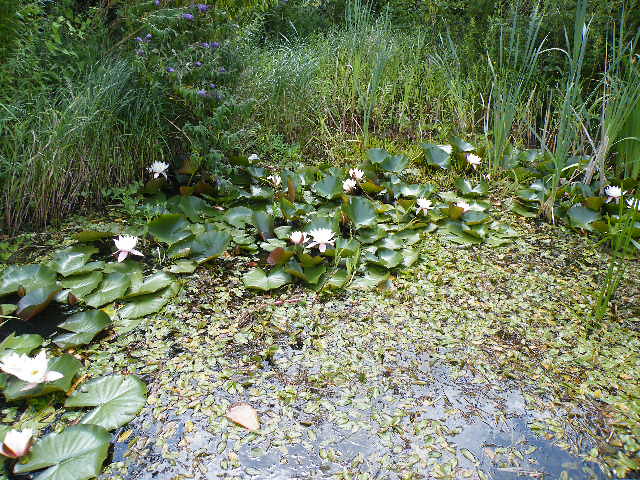This outdoor photograph features a lush, verdant scene dominated by a variety of greenery and an overgrown water body. In the lower center foreground, a puddle of murky, dark water is adorned with large, green water lily leaves and blooming white water lily flowers, some with a yellow center. These lilies form an arching pattern from the lower left to the upper right. The water appears swampy, filled with vegetation, and occasionally dotted with what look like dead water lilies. Surrounding this water feature, possibly a pond or a very stagnant body of water, is a landscape of tall green grass and various shrubs reaching heights of three to four feet. In the background, the dense foliage of trees and bushes creates a natural, wild backdrop, hinting at untamed growth and a thriving ecosystem.